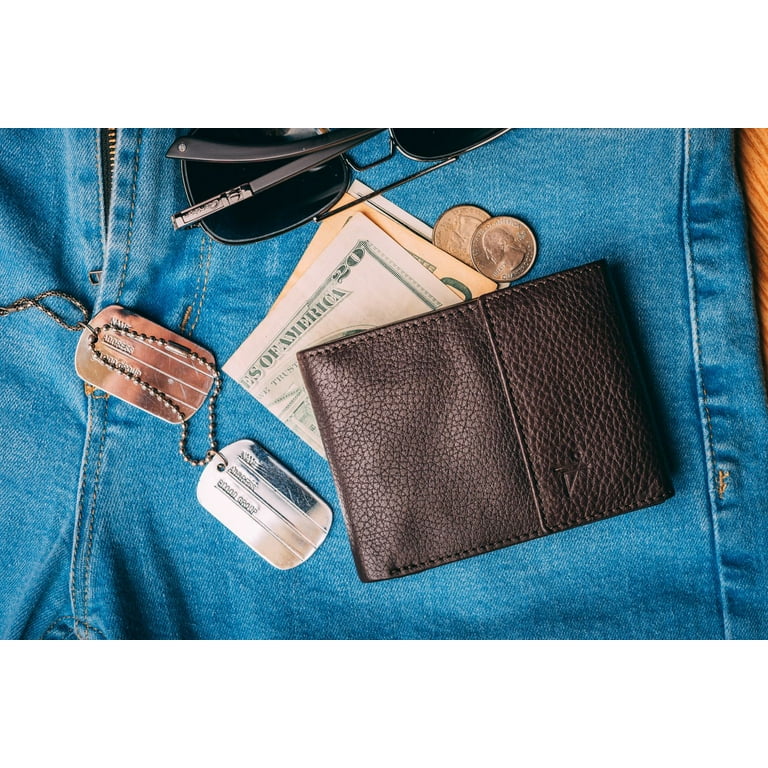The image depicts a meticulously arranged set of items placed on a pair of blue jeans, resting on a wooden surface that is visible as a sliver in the background. The focus is on the upper section of the jeans, primarily around the area of the zipper, creating a visually pleasing composition.

On the lower right of the jeans lies a dark brown leather billfold, featuring a distinct 'V' imprint. Partly protruding from the billfold are some folded $20 bills. Nearby, there are two quarters, one showing its obverse side while the other displays its reverse. Positioned above the wallet is a pair of stylish black aviator sunglasses with gray sides, crossed over in a leisurely manner.

To the left of these items, a set of dog tags rests, suspended from a single chain. One tag is silver and the other exudes a coppery gold hue, adding a touch of contrast to the overall scene. The entire arrangement conveys a sense of modern, casual sophistication, neatly laid out on the classic blue denim.